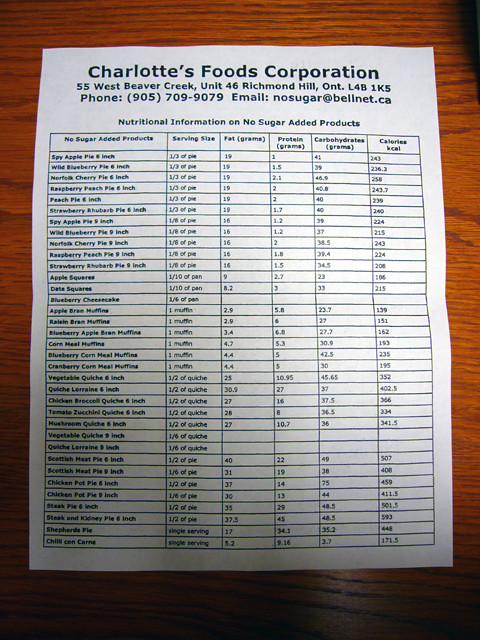The image depicts a white piece of computer paper with black text, resting on a finished brown wooden table. At the top, it reads "Charlotte's Foods Corporation" followed by the address "55 West Beaver Creek, Unit 46, Richmond Hill, Ontario, L4B 1K5". Below this, the company's phone number "905-709-9079" and email address "nosugar@belknet.ca" are provided. The document is titled "Nutritional Information on No Sugar Added Products" and features a detailed table with six columns. These columns are labeled "No Sugar Added Products", "Serving Size", "Fat (Grams)", "Protein (Grams)", "Carbohydrates (Grams)", and "Calories (Kcal)". The leftmost column, which is the widest, lists various no sugar added products such as fruit pies, squares, cheesecakes, muffins, quiches, and pot pies. The table meticulously displays nutritional information for each product.